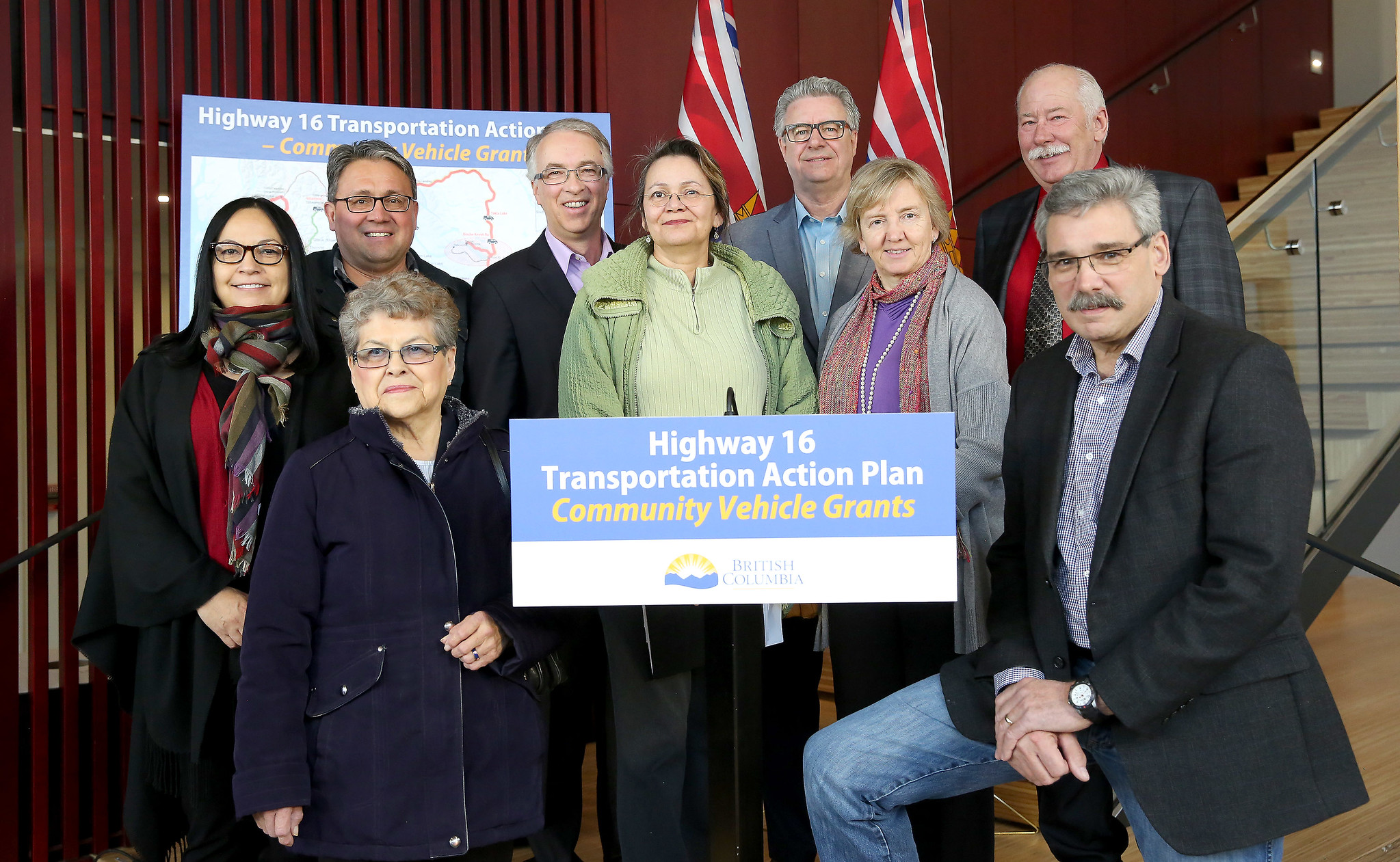In this color photograph, a group of nine older adults, comprised of five men and four women, all Caucasian and dressed formally, pose in front of a red wall adorned with bars and two vertically-hanging flags featuring red and white stripes. Central to the image is a rectangular signboard in blue and white hues. The sign prominently displays the text "Highway 16 Transportation Action Plan" and "Community Vehicle Grants" in white and yellow letters on blue and white backgrounds respectively. Below this, on a white background, it reads "British Columbia" next to a yellow and blue logo. Partially visible behind the group is another notice board that repeats the same text and includes a partially visible map. To the right of this scene, a stairway ascends, adding depth to the setting. The atmosphere suggests a formal but communal gathering, potentially in a government or public service building in British Columbia.